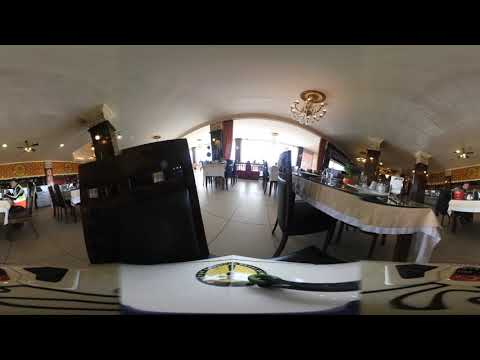The image captures a wide-angle view from a camera atop a vehicle within a spacious restaurant setting. The vehicle occupies the foreground, showcasing its distinct coloration: darker tan corners on either side and a central white section adorned with a black ring, a central symbol of yellow wings, and what appear to be hands grasping the wings. The room itself features large tan tiled flooring with gray grout and numerous tables scattered throughout, each with tan and white tablecloths. 

Although the room appears large due to the fish-eye lens, the chandelier—a brass and crystal piece—hangs prominently in the center, complemented by ceiling fans visible on both sides of the shot. The dining tables vary in size; smaller ones on the left have multiple seats arranged symmetrically, while larger tables with longer seating can be seen to the right. A slanted mini-house structure seems to be located within the dining area, likely a result of the camera's angle.

A couple of people can be spotted: one gentleman sitting at a table on the left, and another person scattered among the chairs. The overall ambiance is relatively empty, suggesting either a quiet period or preparation for an event. Additionally, a couple of black box-like objects are on the left, and more are positioned towards the right side of the room. Despite the fish-eye effect expanding the room’s appearance, the image precisely reflects the sprawling and largely unoccupied space primarily set up for dining.